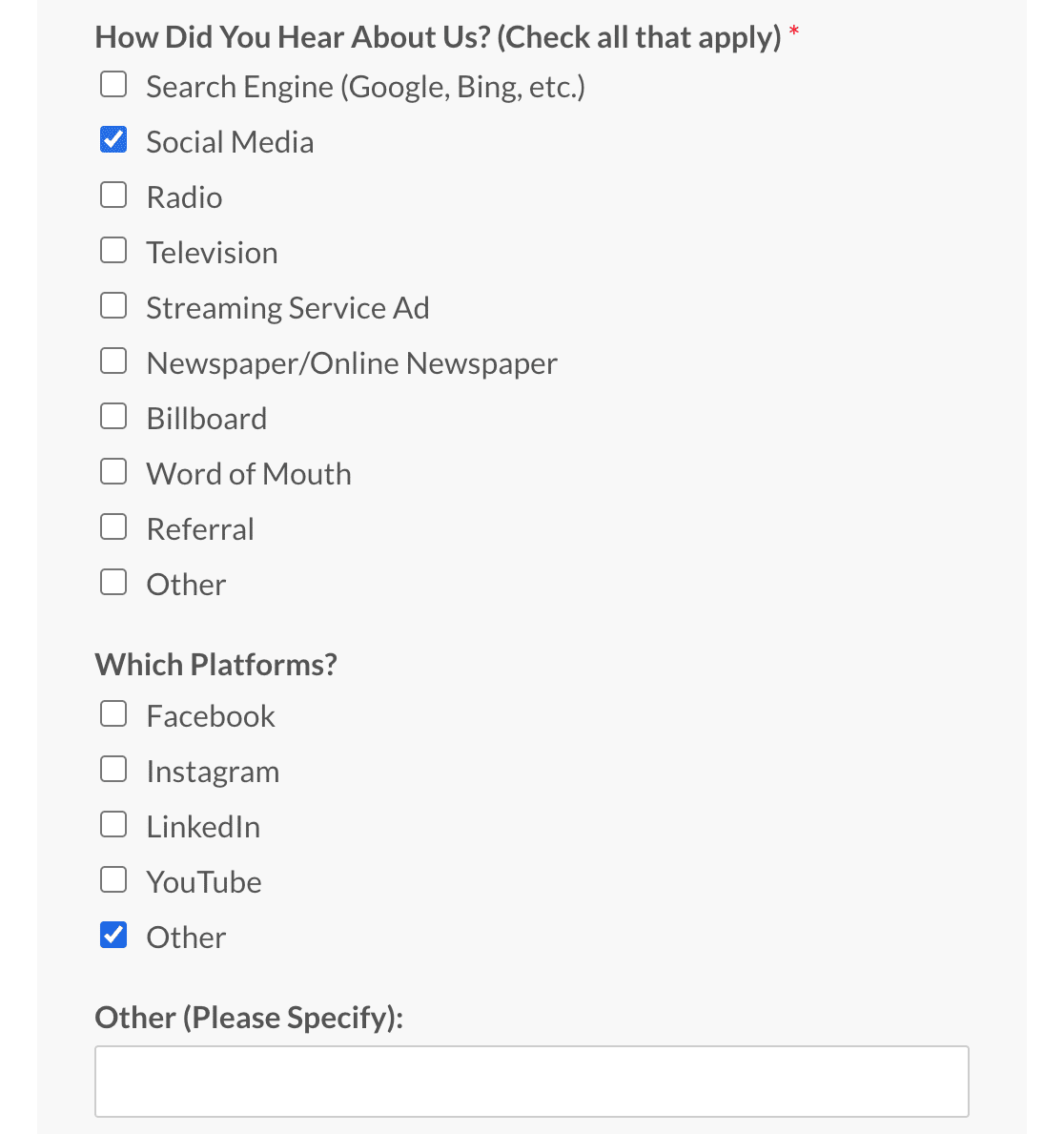The image depicts a website interface designed to gather information on how users discovered the site. The background is entirely gray. At the top of the image, there is a prompt that reads, "How did you hear about us?" followed by a set of instructions in parentheses, "Check all that apply," and a red asterisk indicating that the question is mandatory.

Below the prompt, various options are provided for the user to select. These options include "Search engine (Google, Bing, etc.)," "Social media," "Radio," "Television," "Streaming service ad," "Newspaper," "Online newspaper," "Billboard," "Word of mouth," "Referral," and "Other." Next to each option is a small white checkbox, except for "Social media," which has been selected and thus displays a blue checkbox.

Further down, there is a sub-question labeled "Which platforms?" with corresponding choices: "Facebook," "Instagram," "LinkedIn," "YouTube," and "Other." The "Other" option has been checked, signified by another blue checkbox. Beneath this, there is an elongated input box accompanied by the instruction, "If you checked Other, please specify," in parentheses. Although "Other" has been checked for the platforms question, the user has not yet provided any additional details in the text box.